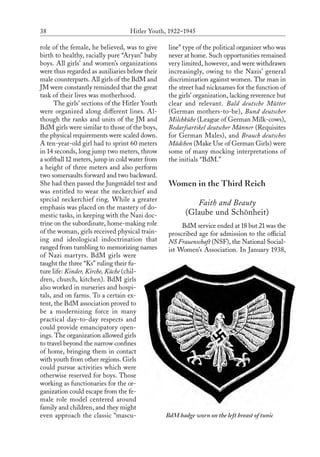This image displays a very detailed page from a book, magazine, or newspaper, identified as page number 38. The page is divided into two columns of text, which are difficult to read due to their small size. In large black letters across the center, the header reads "Hitler Youth 1922-1945." In the second column, towards the bottom right, bold text states "Women in the Third Reich" followed by the subheading "Faith and Beauty," with approximately four lines of smaller, unreadable text underneath. Additionally, there is a significant emblem featuring a black shield with a silver eagle, wings spread wide, and sporting a swastika at its center.